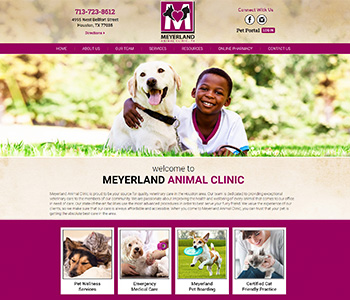**Caption:** 

"Welcome to Mayer Land Animal Clinic"

The image captures a heartwarming scene of a joyful young Black boy laying on the grass with his arm lovingly wrapped around a white dog sporting a black collar. The boy, who has short black hair, is dressed in a white shirt with a red collar and holds a blue retractable leash, giving the dog some freedom. Both child and dog exude happiness, with the boy flashing a broad smile. In the background, lush trees complete the serene setting.

Above this touching scene, the text reads "Maeve, Mayer, Land, M" with a heart symbol, accompanied by illustrations of a horse and a cat. 

Below this image, further text reads "Welcome to Mayer Land Animal Clinic," followed by four separate smaller images: 
1. A dog and cat peacefully sleeping together on a bed.
2. A person holding a dog while another individual handles a pink roll of tape.
3. A dog mid-air catching a blue frisbee.
4. A smiling white woman in a gray sweater holding a white cat on her leg; the cat appears slightly grumpy.

For more information, visit [YouTube link] or check the description below.